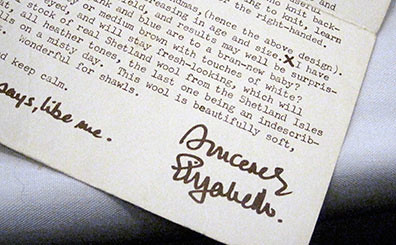This image depicts the corner of a typewritten letter that appears to have been folded, likely for placement in an envelope, and then unfolded. The text of the letter, which is partially readable, seems to discuss fabrics or textiles—perhaps related to fashion—mentioning specifics like "hence the above design" and phrases like "increasing in age and size." The visible content includes mentions of "pink and blue are to a brand new baby," albeit "brand" is misspelled, and "medium brown touches of white." Another fragment notes, "we'll stay fresh-looking, which will stock of real Shetland wool," and praises the wool as "beautifully soft, wonderful for shawls." The letter finishes with a signature in the bottom right corner, written in large, bold black Sharpie, although the name is indiscernible. The letter is laid on a gradiated background that transitions from white to gray, possibly resting on a denim surface. Handwritten annotations include a notable 'X' and a partially legible note stating, "keep calm, like me, sincerely."